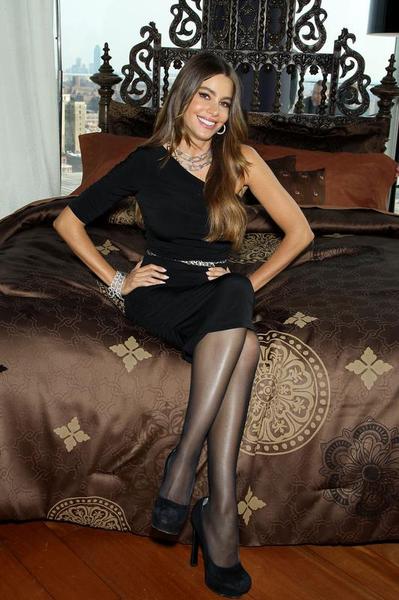The image features actress Sofia Vergara sitting on a luxurious brown bed adorned with abstract flowery designs on its comforter. The bed is detailed with large bedposts and a substantial head frame. Positioned directly in the middle of the image, Sofia is smiling at the camera, with her hands on her hips, forming a triangle shape with her arms. She is wearing a sophisticated black dress, which is sleeveless on her left arm and features a medium sleeve on her right arm. Her accessories include a silver belt around her waist, hoop earrings, a chain necklace, silver bracelets, and black high heels paired with pantyhose leggings. The background showcases a large window framed by a white curtain, offering a view of a distant city skyline against a blue sky. The room has red wooden floorboards, and there are pillows resting against the headboard—two small ones in brown pillowcases and two larger ones in red cases. There's a hint of an elaborate table or sculpture at the headboard’s end, and a man is partially visible just at the right side.